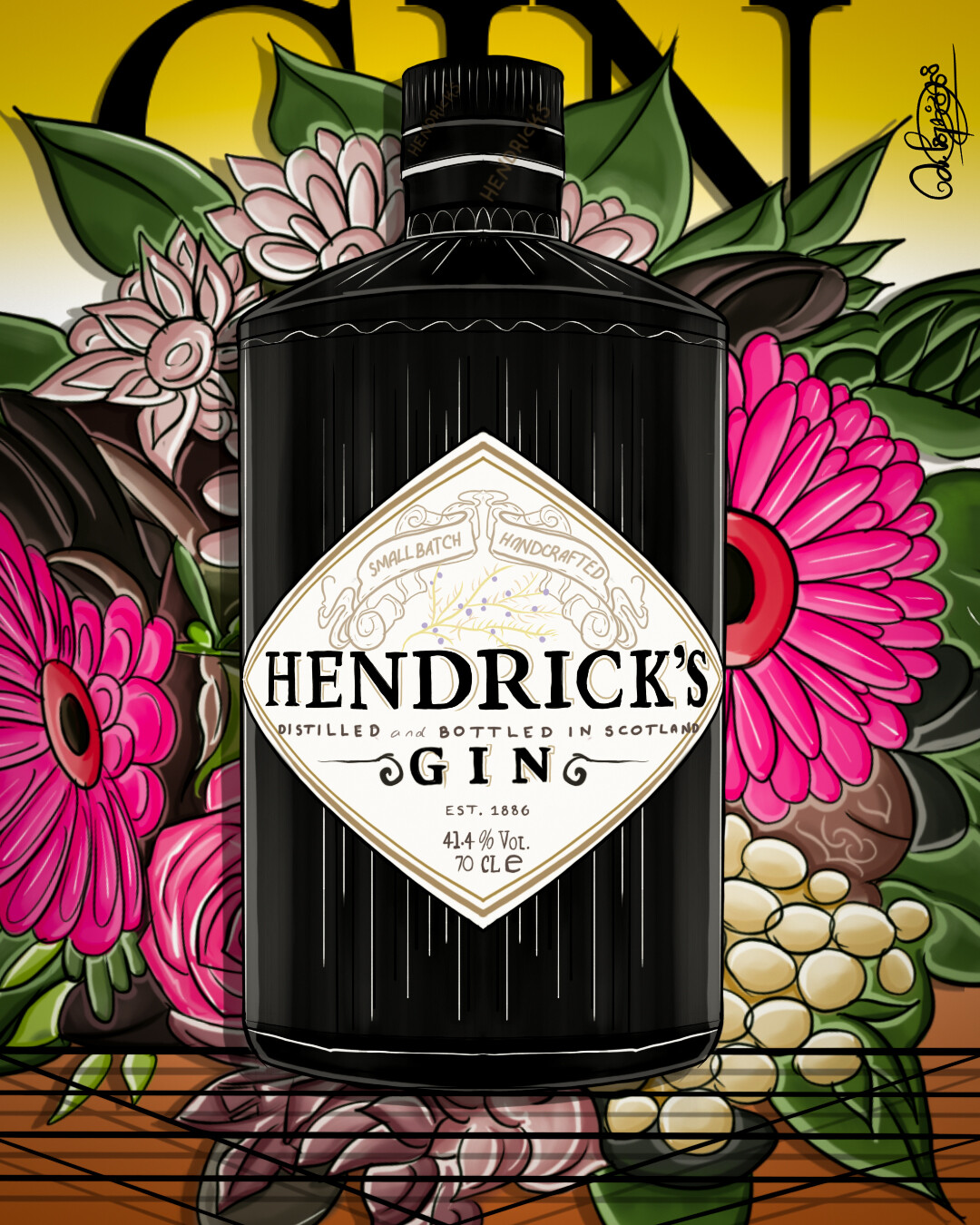The image is a detailed, hand-drawn advertisement for an alcoholic beverage—specifically, a black cylindrical bottle of Hendrix Gin. The bottle features a black twist top and a prominent white diamond-shaped label with a gold border. At the top of the label, two gold banners read "Small Batch Handcrafted." The central portion of the label boasts large black text that reads "Hendrix." Below this, in brown text, it says "Distilled and Bottled in Scotland," with additional details at the bottom corners of the diamond such as "Established 1886," "41.4% Volume," and "70 CLE." 

Behind the bottle, the background transitions from yellow to white vertically and is adorned with an illustration of various flowers—primarily pink, but also including purple and yellow blossoms, amidst green foliage. The word "Gin" in large black letters can faintly be seen in the background, partially obscured by the floral illustrations, giving depth to the overall advertisement.